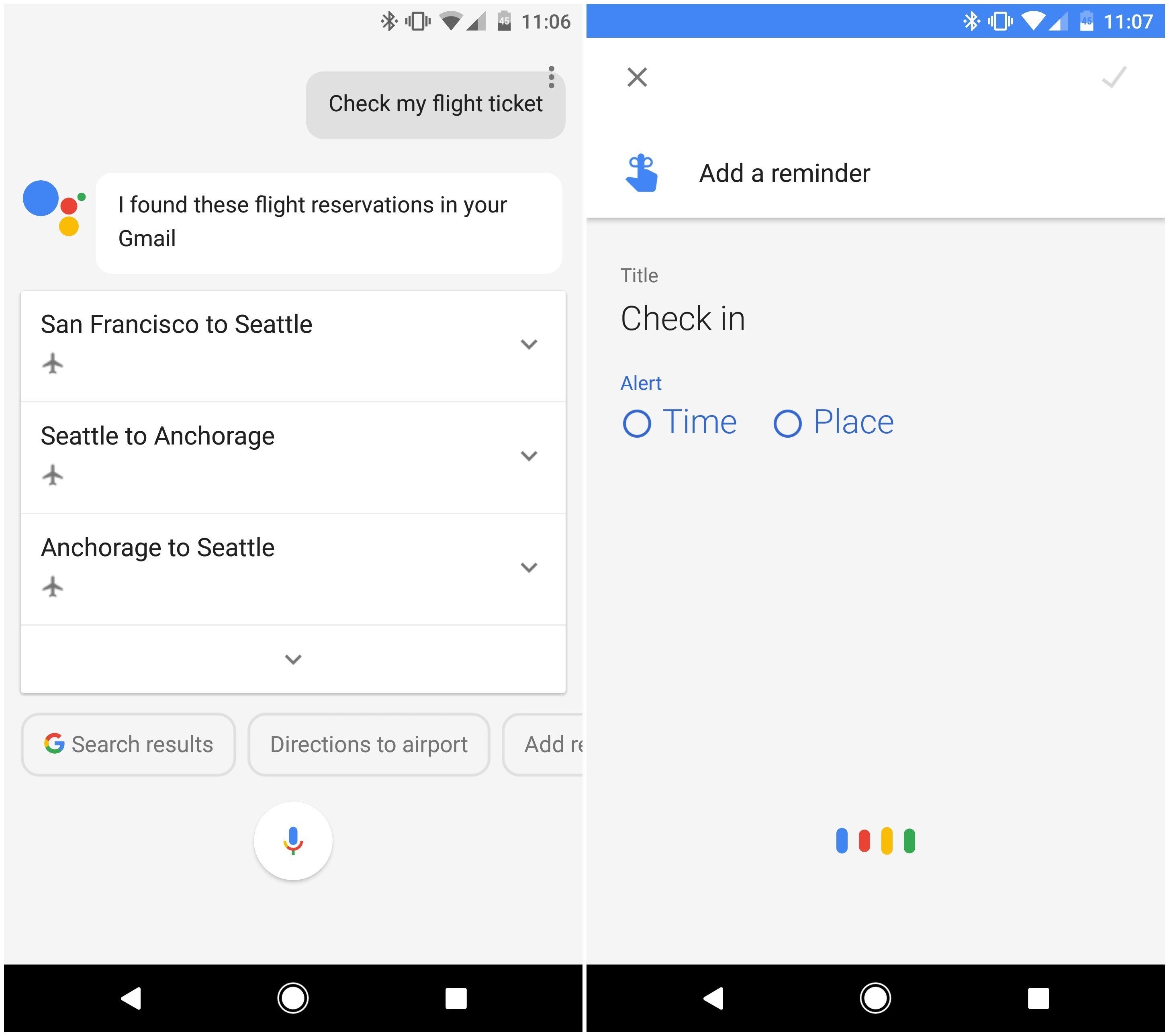A composite image of two side-by-side mobile screenshots, both displaying elements of a Google application interface. 

The left screenshot, stamped with the time 11:06 in the upper right corner, includes standard phone status icons such as battery percentage, cell signal, and Wi-Fi strength. Below these, it features a search query, "check my flight ticket," accompanied by Google's automated response: "I found these flight reservations in your Gmail." Three expandable menus follow, detailing flight segments from San Francisco to Seattle, Seattle to Anchorage, and Anchorage to Seattle, respectively. Options for further actions are provided, including searching results and getting directions to the airport.

The right screenshot, marked at 11:07 in the same indicator section, mirrors the left but is distinguished by a blue header bar indicating the ability to set flight reminders. This screen offers additional functionalities such as "check in," and options to set alerts based on specific times or locations.